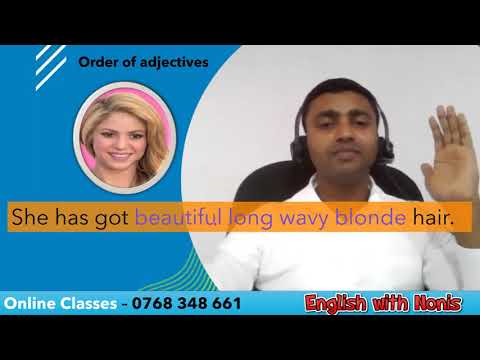The image is an advertisement for online classes that features a dark-skinned Indian man with short, dark hair, wearing over-the-ear black headphones and a white button-down shirt. He is seated in a black office chair, facing the camera with his left hand raised, palm facing out, as if swearing an oath, and displays a serious expression. The background is predominantly white, with an overlay design. 

To the left of the man, there is a blue background with rounded borders, which includes a circular thumbnail image of a smiling Shakira against a pink backdrop. Above the thumbnail, black text reads "Order of Adjectives." 

An orange banner spans the full width of the image near the center, featuring the text "She has got beautiful long wavy blonde hair." At the bottom of the image, there is a black bar that contains the text "Online Classes - 0768-348-661" on the left and "English with Nonnies" on the right.